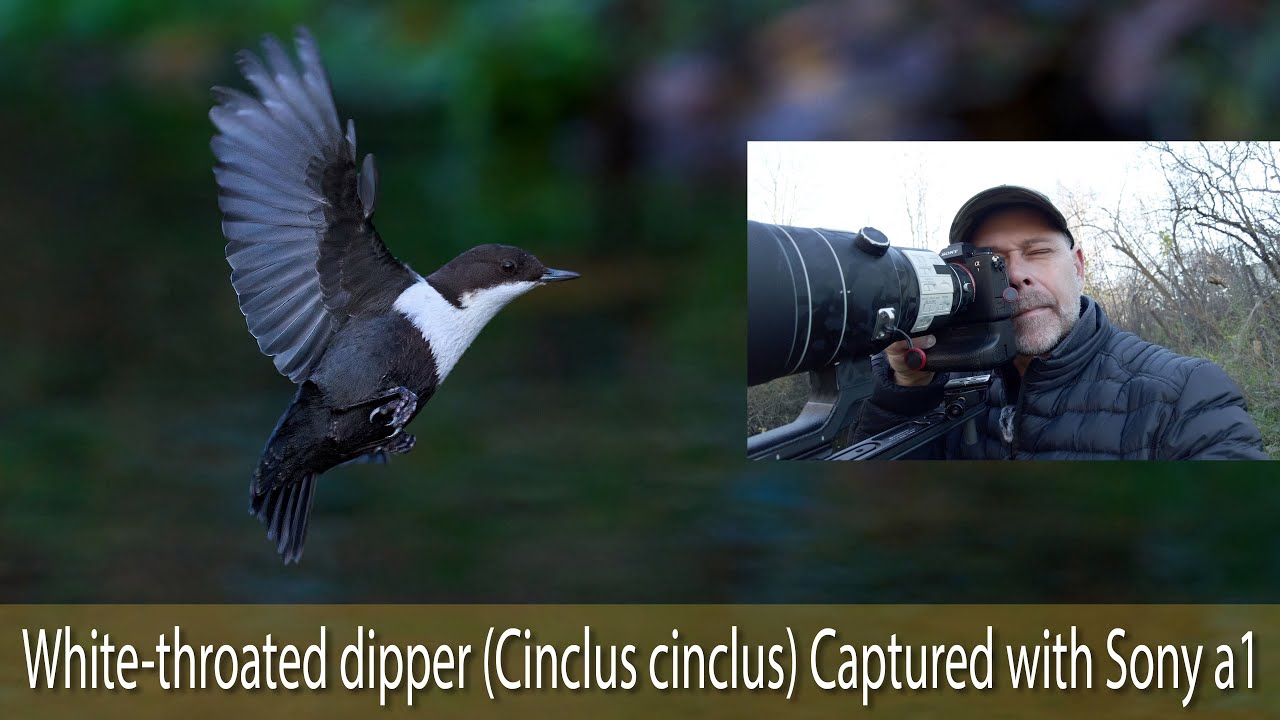This captivating image is a detailed composite featuring two superimposed photographs. The larger, background photo showcases a white-throated dipper (Cinclus cinclus) in mid-flight against a blurred, forested backdrop with hues of green, brown, and blue. The bird is mostly black, including its beak, eyes, and feet, except for its distinctive white throat and underbelly. Its wings are spread wide, captured with extraordinary clarity, suggesting the use of a high-speed lens, indicative of advanced wildlife photography techniques. At the bottom of this larger photo is a gold banner with the text "Captured with a Sony A1."

Superimposed on the right side of the larger image is a smaller, crisp photograph of the photographer: a middle-aged, light-skinned man with a gray beard. He is dressed in a black puffer winter jacket and a cap, intently looking through the viewfinder of a large camera with an exceptionally long lens, presumably the Sony A1. This juxtaposition of images not only highlights the detailed capture of the white-throated dipper in mid-flight but also pays homage to the skill and equipment of the dedicated photographer who achieved this remarkable shot.